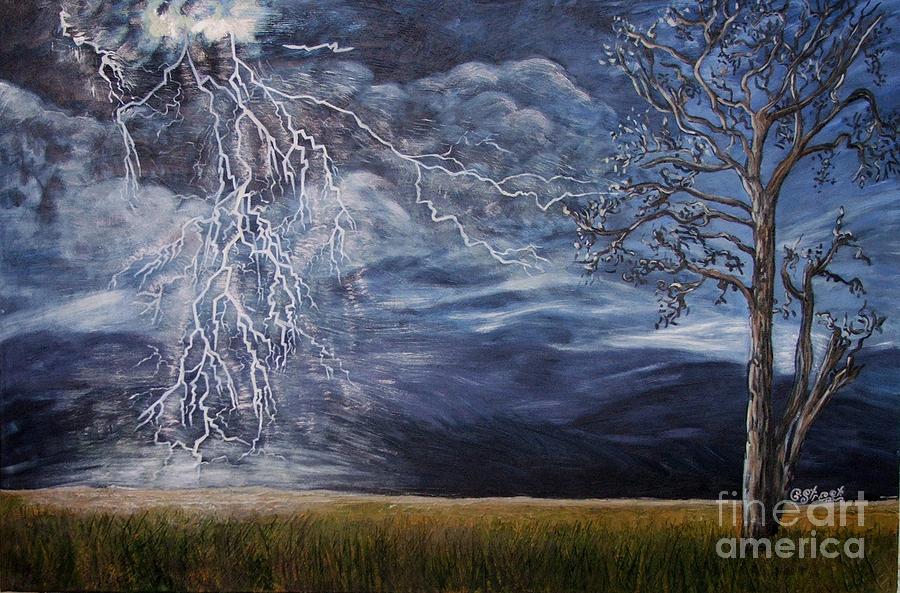The painting, likely sold by Fine Art America, showcases a dramatic stormy night over an empty farmland, rendered in an impressionist style, possibly using oil paints. Dominating the scene is an intense, vivid lightning strike branching out from a bright cloud on the top left. The lightning's splintered paths stretch across the dark, tumultuous sky filled with swirling grey, black, and hints of blue, indicating a fierce storm without visible rain. Brush strokes suggest wind movement flowing from left to right. At the bottom right stands a tall, dry tree beside a field of knee-high, bright green grass. The eye-catching contrast between the lightning and the dark sky draws immediate attention, evoking a powerful, almost palpable sense of the storm's intensity.